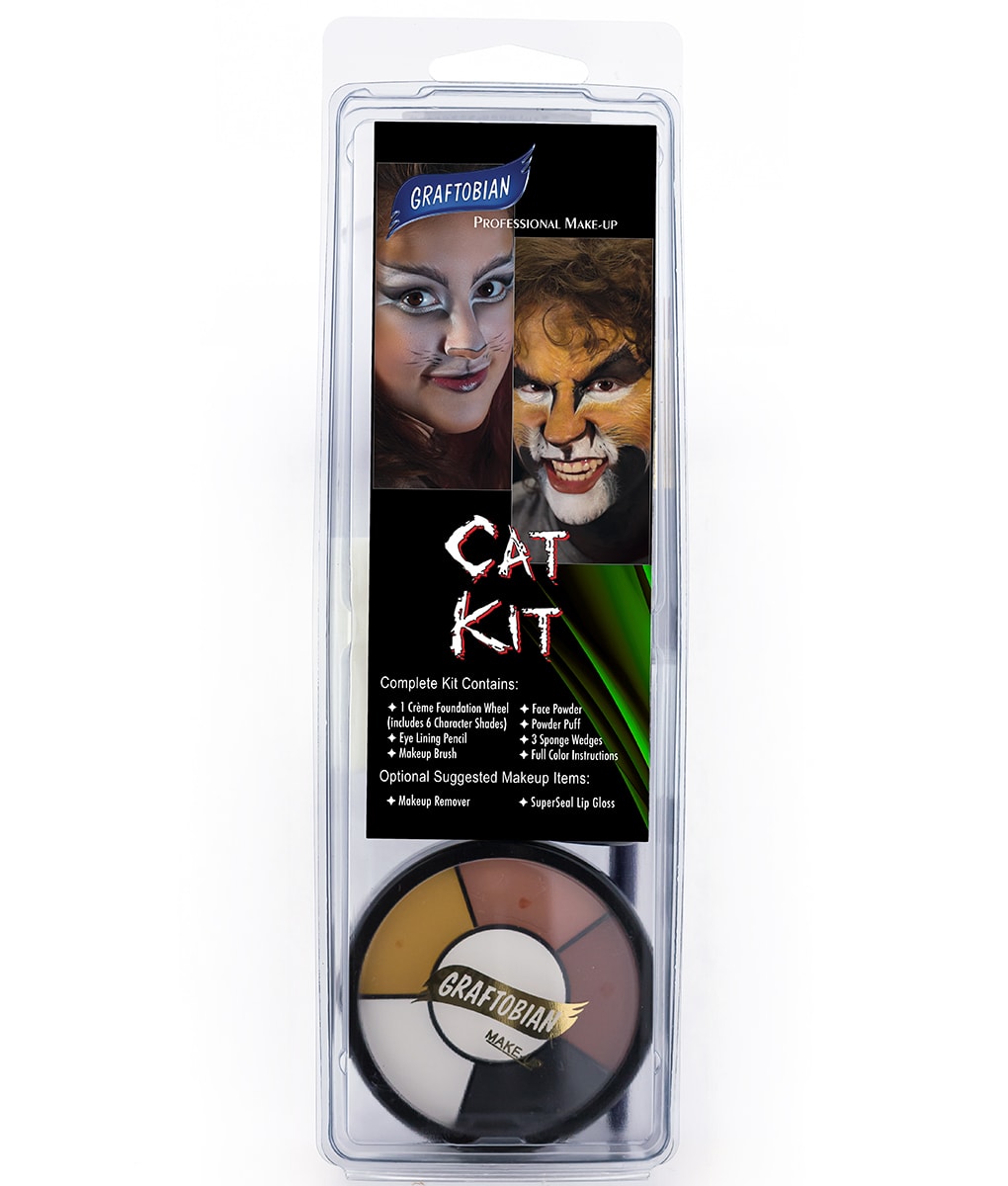This image portrays a vertical, rectangular professional makeup kit encased in plastic, prominently featuring the brand name "Graftobian" in white lettering against a blue banner at the top. The center of the kit reveals the bold white letters "Cat Kit" on a green background, indicating its thematic design for creating cat-like facial transformations. Adjacent to this text are two visual examples: on the upper left, a woman adorned with detailed cat whiskers, eyelashes, and red lipstick, and to her right, a man with an intricately painted cat face in shades of orange, white, and black.

Below the central "Cat Kit" title, the kit lists its complete contents, which include one cream foundation wheel with six character shades, an eyelining pencil, a makeup brush, face powder, a powder puff, and three sponge wedges, all accompanied by full-color instructions. Optional suggested items such as makeup remover and super seal lip gloss are also mentioned. At the bottom of the kit is a circular section holding the makeup wheel, featuring colors like orange, white, black, and two shades of reddish pink, bounded by the Graftobian logo in white on a black background.